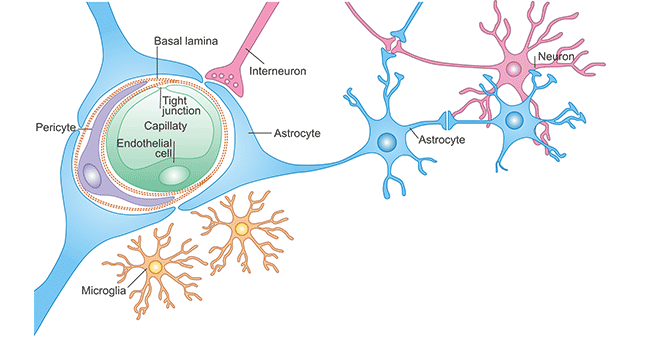This scientific or medical illustration, set against a white background, depicts intricate neural and cellular structures in the brain with various colors highlighting different components. On the left side of the wide, horizontal diagram, a large light blue structure with three branching extensions is prominent. The top left branch extends upward to the corner, the lower left branch reaches to the lower corner, and the center branch stretches towards the upper right. Inside this blue structure, several concentric circles are colored white, purple, yellow-orange, dark green, and a lighter green at the center. 

Within these circles, black text with arrows identifies critical elements: "Basal Lamina" in the purple circle, "Tight Junction," "Capillary," and "Endothelia Cell" in the green circles. An orange dotted line encircles this region. 

Extending from the blue structure is a pink branch labeled "Interneuron," along with various non-attached blue and gold spidery circles indicating "Astrocytes" and "Microglia," respectively. The blue blob itself is denoted as an "Astrocyte." Additionally, black text on the left side identifies "Pericyte," further detailing the cellular makeup. This detailed labeling and color-coding emphasize the complex interactions and structures within the brain.